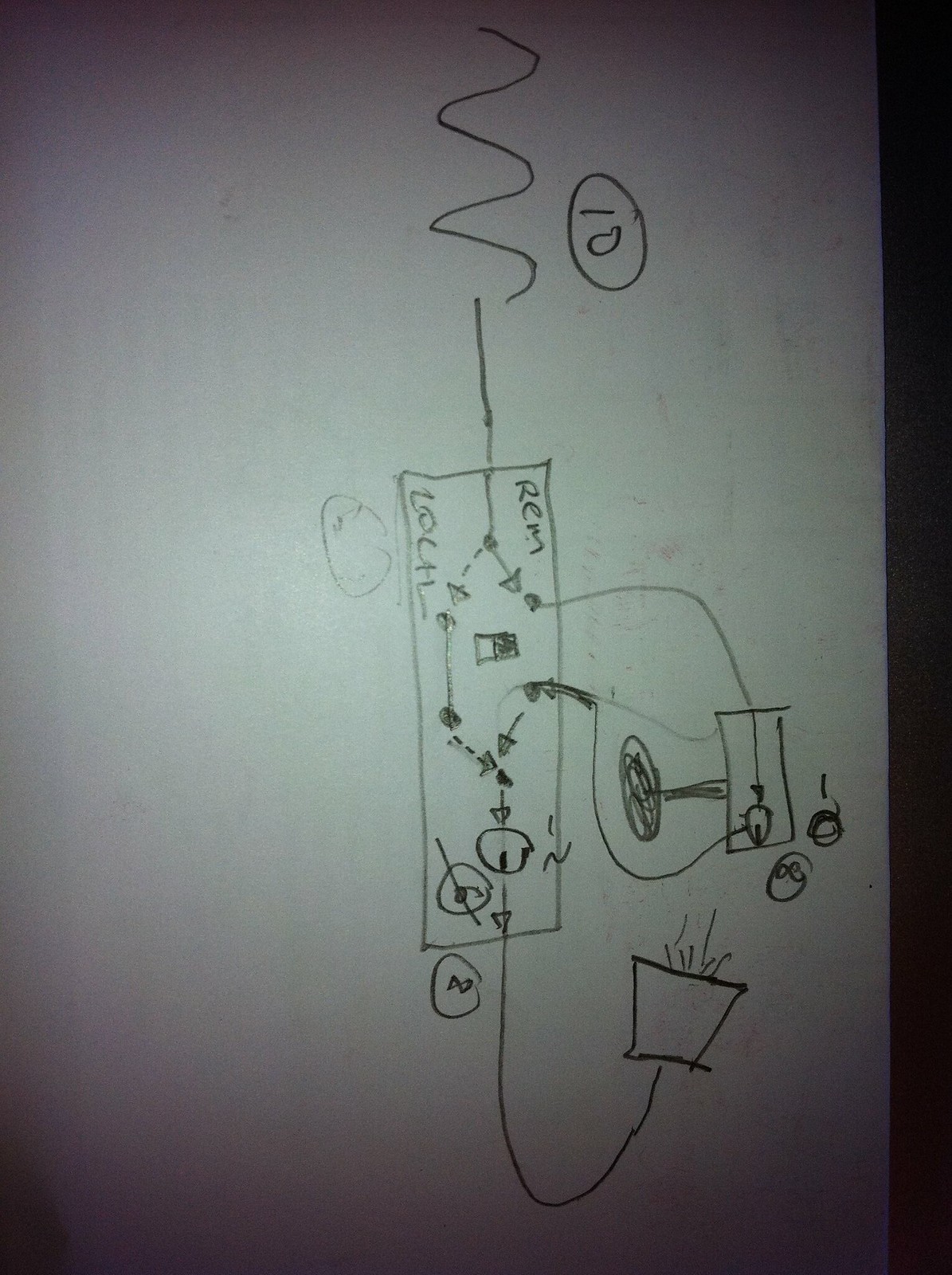This photograph features a design document placed against a dark background, likely captured with a camera flash, which causes a bright glare in the center and shadows along the top and bottom edges. The drawing at the top of the page depicts a squiggly line resembling half of a DNA helix, descending vertically into what appears to be a wire.

This wire connects to a rectangular device that resembles a remote control. The device is oriented upside down and covered with various buttons. Notable text is visible at the top corners of the device: "REM" on the top right and "Local" on the top left. The entire drawing is rendered in black and white, with no additional colors.

At the bottom of the page, the wire extends towards what looks like a wall outlet, suggesting that the device can be plugged in. On the right side of the drawing, two wires lead to another device. This secondary device has a protruding object that looks similar to a doorknob, emerging from its left side, and connects into another rectangle.

This detailed sketch appears to represent a circuit or a device setup, potentially for an electronic or control system.